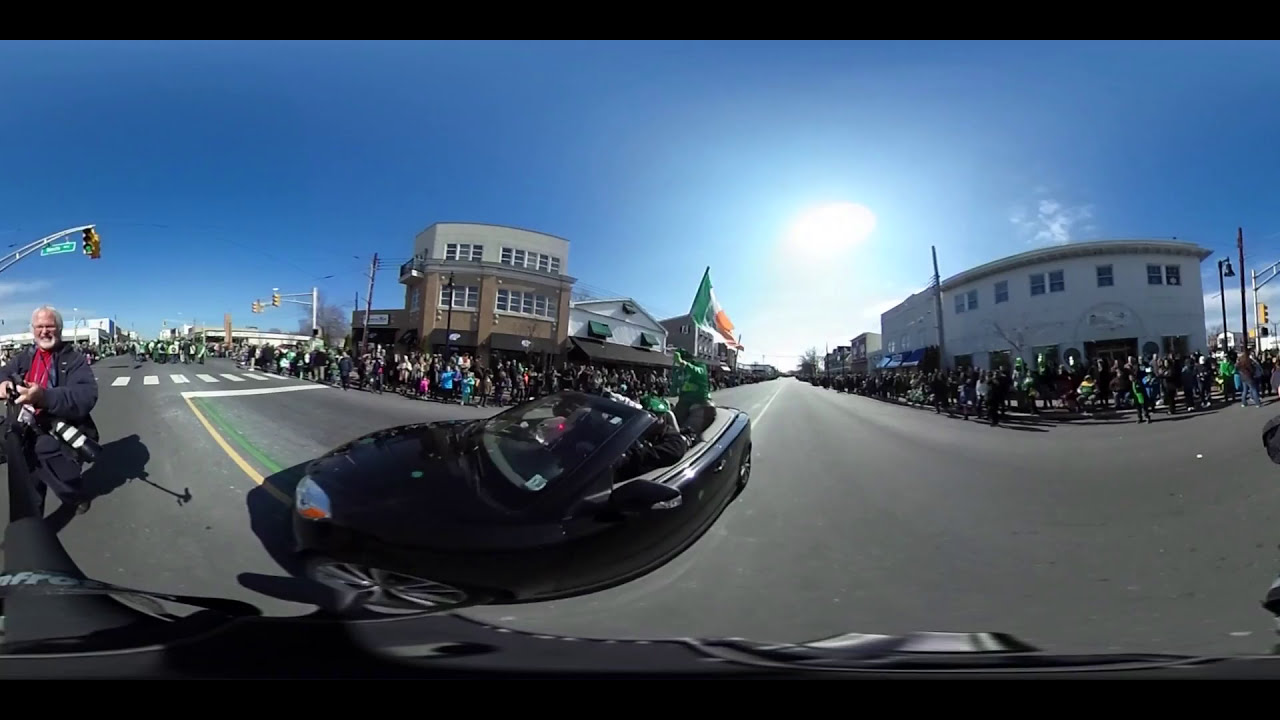The image captures an outdoor scene, likely at a parade, viewed from inside a vehicle on the street. In the foreground, a black convertible appears unnaturally bent, possibly due to lens distortion. Someone is seated in the trunk area of the convertible, waving. The left side of the image showcases a tan and brown three-story building, where a crowd of people stands on the sidewalk, suggesting a festive gathering. Among them is an elderly man with gray hair, a gray beard, and sunglasses, wearing a red shirt and black jacket. He stands near the left center of the image, under a streetlight and a green traffic sign, with a crosswalk nearby. On the right side, another building, which has a rounded facade with five windows on the upper level and a storefront below, is also flanked by a crowd. Above, the sky is bright blue, complementing the vibrant street scene.